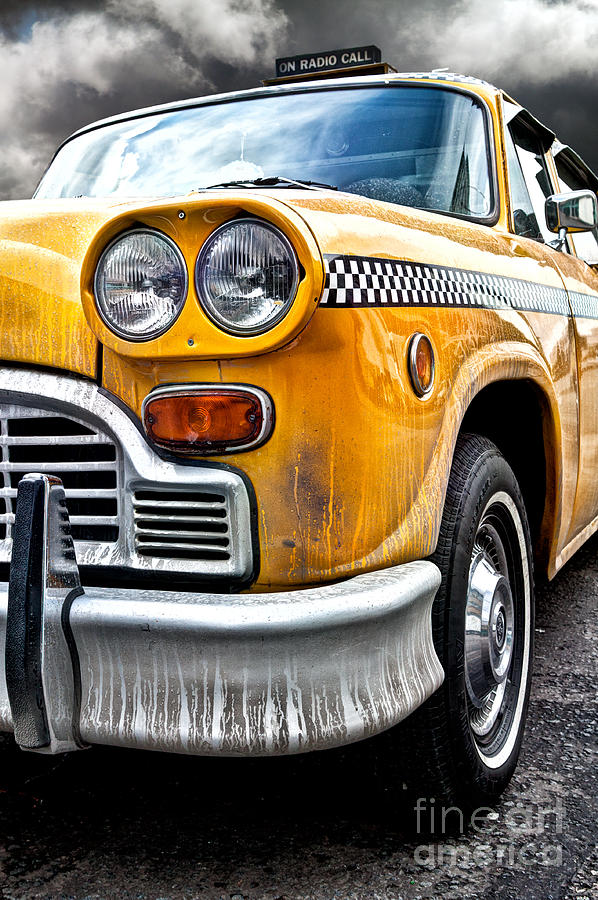This detailed close-up image captures an old-model yellow taxi cab, characterized by a slightly orangish hue. The taxi, partially shown from the front and side, features a distinctive black and white checkered stripe along its side. The vehicle appears dirty, with noticeable dust and mud, and stands on a grey surface. Its black tires and a visible front grill add to the vintage feel. Atop the taxi, a black sign with white letters reads "ON RADIO CALL." The sky above looms dark and gray, with patches of light grey clouds, creating an ominous atmosphere. Additionally, a watermark in the bottom right corner identifies the image with "Fine Art America," suggesting it might be an artist's rendition rather than an actual photograph.